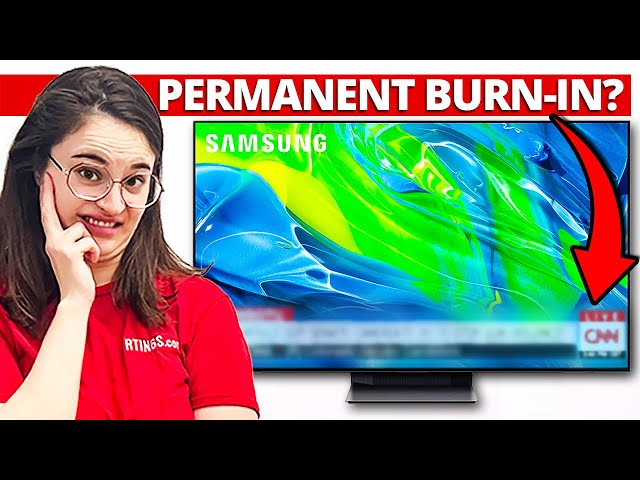In this horizontally aligned, rectangular image, a young Caucasian woman in her 20s stands to the left of a large Samsung television screen. She's wearing large, hexagon-shaped glasses and a red t-shirt with some sort of illegible white writing due to the wrinkles in the fabric. The woman has shoulder-length, straight brown hair and is adorned with pink lipstick. Her expression is one of concern or confusion, with her eyes raised, creating wrinkles on her forehead, and her right hand partially covering her face as if she's contemplating something. Her two fingers rest on her cheek while the other two are placed near her chin.

The television screen next to her displays a live CNN broadcast, indicated by the CNN logo in the lower right corner. The screen is filled with vibrant blues, greens, and whites, giving it a dynamic look. Above the TV, there is a prominent red banner reading "PERMANENT BURN IN?" with a large red arrow pointing downward toward the CNN logo. The image appears to have originated from a TV review, possibly a screenshot from a YouTube video by the website Rtings.com. At the top and bottom of the image are black letterbox bars, contributing to the appearance of a screenshot.